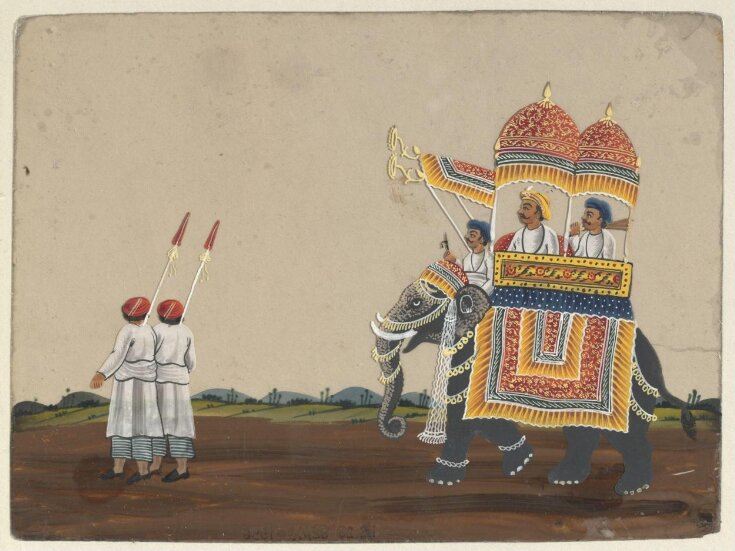This hand-painted illustration depicts a richly adorned Indian scene. The central focus is a grand, gray elephant adorned with an elaborate rectangular blanket featuring an orange border, intricate blue designs, and red floral motifs. The elephant is further embellished with ornate jewelry around its head, trunk, and ankles. On its back, a lavishly decorated carriage, covered by two red and gold domes with pointed tops, houses two officials. In front of the carriage, a third man sits under a small canopy, likely controlling the elephant. Leading this majestic procession are two footmen dressed in white robes, red hats, striped pants, and shoes, each holding a spear. They walk on a brown dirt road which extends into a distant green landscape. The sky overhead, covering about two-thirds of the image, is a simple, tannish gray expanse, suggesting it's painted directly onto the same textured material as the rest of the scene.